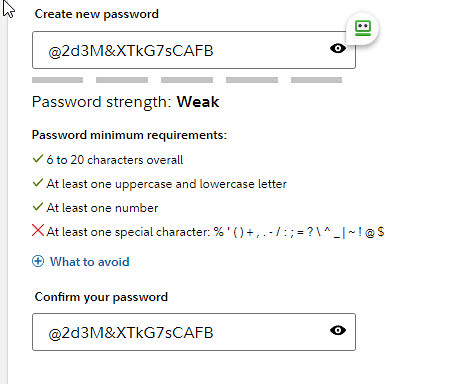This square image features a digital password screen on a white background. The left side of the image is marked by a thin, light gray rectangle running vertically down the entire image. At the top right, bold black text reads "Create New Password." Directly below this, a wide black rectangle filled with white displays the password "2D3M XTKG7SCAFB," along with an eye symbol to the right for revealing the password. Below this, the screen shows five gray rectangles in a row, indicating the password strength as "Weak."

Under the strength indicator, the text outlines password minimum requirements, listing "6 to 20 characters overall," "at least one uppercase and lowercase character," "at least one number," and "at least one special character." The first three requirements are met, indicated with check marks, but the special character requirement shows a red "X." Additionally, there is blue text that reads "What to Avoid," followed by sections for expanding details and confirming the password.